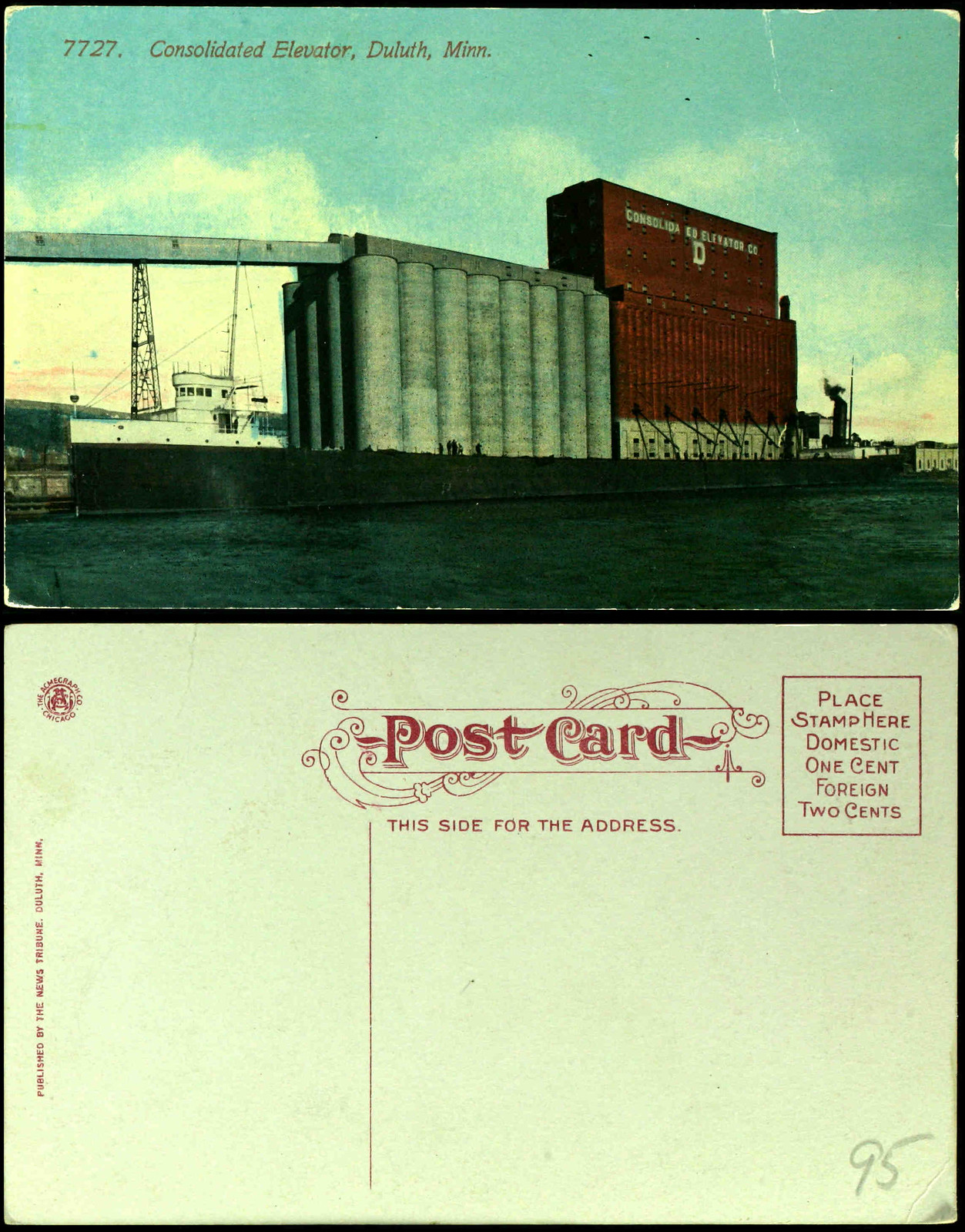This vintage postcard features a long, black-hulled cargo ship with the text "Consolidated Elevator 7727, Duluth, MINN" in the upper left corner. The ship, which appears more like a barge, has a white cabin and stands against a background of blue sky and clouds. At the center of the vessel, silver spiral canisters – possibly metal silos – rise vertically, with a conveyor belt descending to the left from their tops. Behind these canisters, storage containers are stacked, including two dark red ones and a yellow container underneath.

Both the front and back of the postcard are displayed in the image. The front of the postcard, showing the ship, has a somewhat washed-out and murky color palette, indicative of age. In the upper left corner, there is additional white text reading "Consolida EU Elevator Company." The back of the postcard, which has a yellowed appearance, features elaborate floral designs surrounding the red text that reads "Postcard." Instructions for addressing the postcard are specified below, directing "this side for the address" and indicating postage rates with "place stamp here, domestic one cent, foreign two cents" in a red-bordered square. There's also a small emblem in the left corner and a grey number "95" in the bottom right. Additionally, vertical red text, too small to decipher, runs along the left edge. This postcard was published by the News Tribune in Duluth, Minnesota.